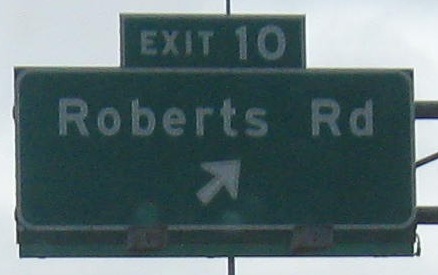This image appears to have been taken from the perspective of a road, looking up at a highway street sign against a whitish-gray sky. The focal point is a large green rectangular sign supported by cylindrical poles visible to the right. The sign features a white-lined border and reads "Roberts Road" with a white arrow pointing upward and to the right. Above this primary sign, there's a smaller green rectangular sign with a similar white border that reads "Exit 10." Additionally, a cylindrical dark-colored shape runs vertically from the top to the bottom of the image, likely another structural support element for the signage.